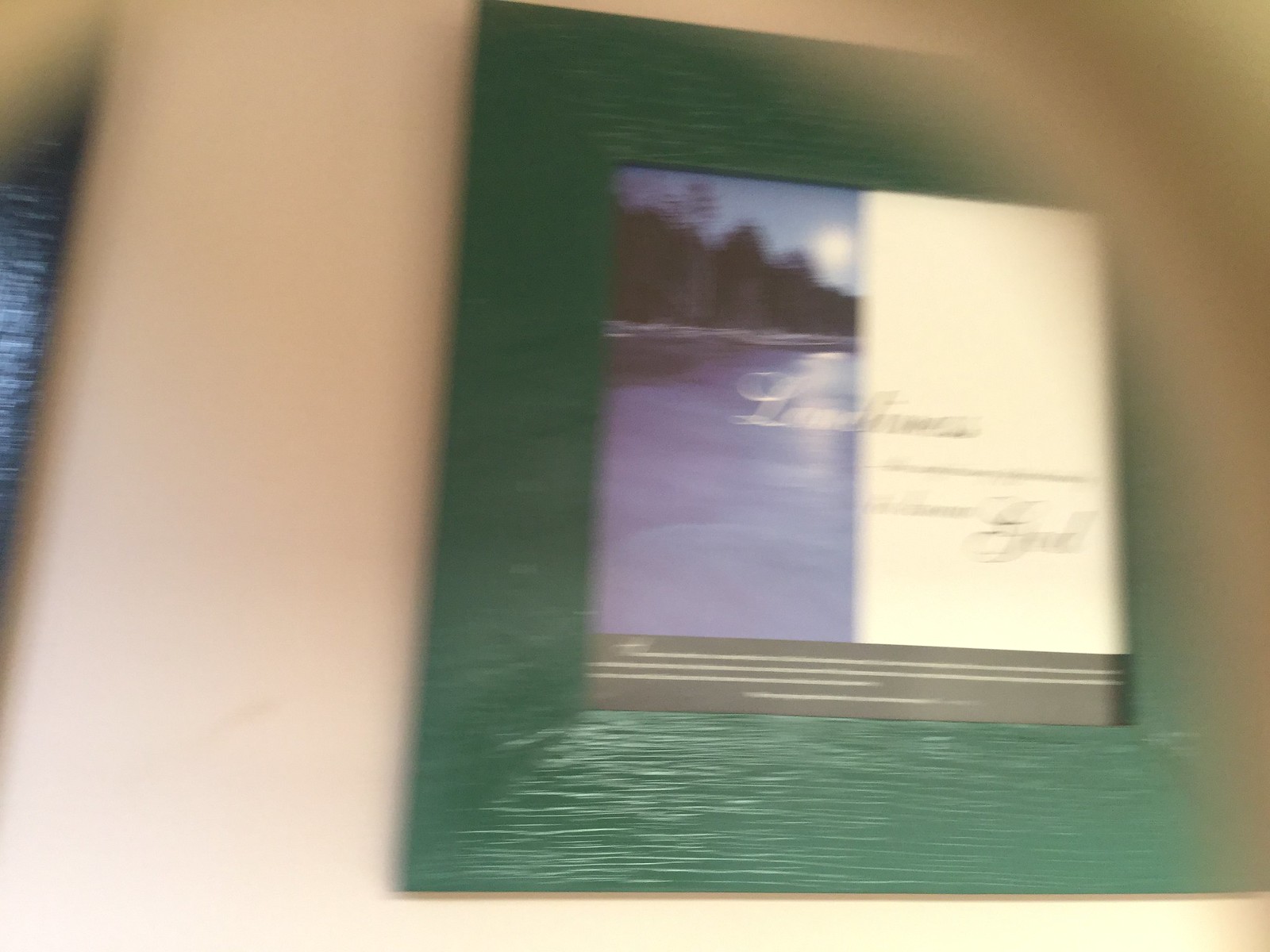The image is a low-quality and somewhat blurry real-life photo, appearing to be taken with a moving camera. The focus is on a very thick, dark green wooden frame, which outlines a smaller, blurry image inside the frame. The inner image is split into two sections: the left side resembles a coastal scene with water and distant trees, accompanied by a partial blue sky. The right side is a white rectangle containing cursive text which is difficult to decipher but might include the words "lifetimes" or "loneliness" and "good."

The background is a beige or cream color with blue jean-like patches on the left side. In the top right corner, part of the image is obscured, possibly by a finger close to the lens, lending a brownish blurry effect. Overall, the photo is not centered on any specific detail, adding to its unfocused and unclear appearance.